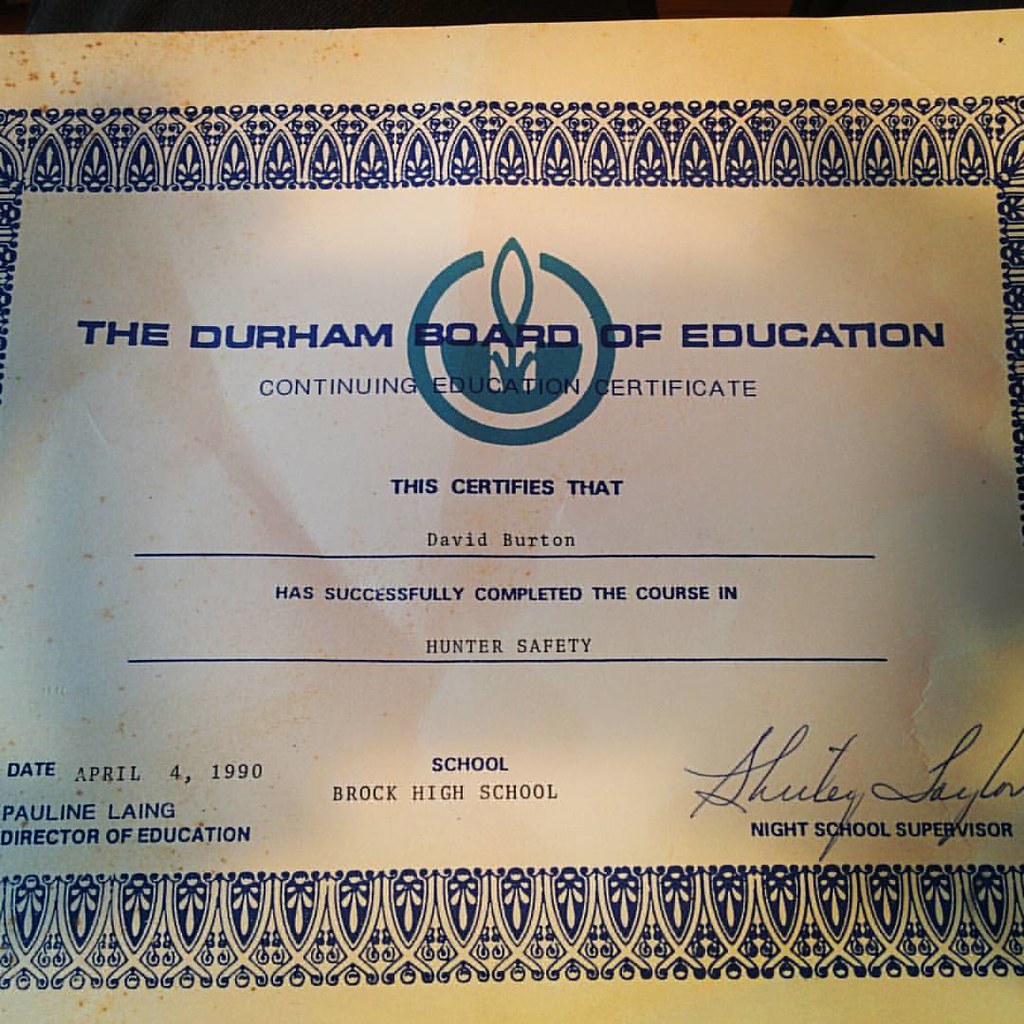The image is of a certificate issued by the Durham Board of Education. It is crafted on light brownish paper, adorned with an elegant blue and white floral design border that frames the document on all sides. The certificate prominently displays "Durham Board of Education" in large blue lettering, with a subtle emblem in the background. Directly below that, in smaller text, is the title "Continuing Education Certificate."

The certificate reads: "This certifies that David Burton has successfully completed the course in Hunter Safety." The recipient's name, David Burton, appears clearly, with a line underneath to emphasize completion. Below this statement, in the bottom left corner, the date "April 4, 1990" is mentioned alongside the name "Pauline Lange, Director of Education." Towards the middle, the name of the institution, "Brock High School," is situated prominently. On the bottom right, there is a handwritten signature attributed to "Shirley Taylor, Night School Supervisor." The intricate blue border design featuring floral elements adds an aesthetically pleasing touch to the certificate, underscoring its significance and formality.